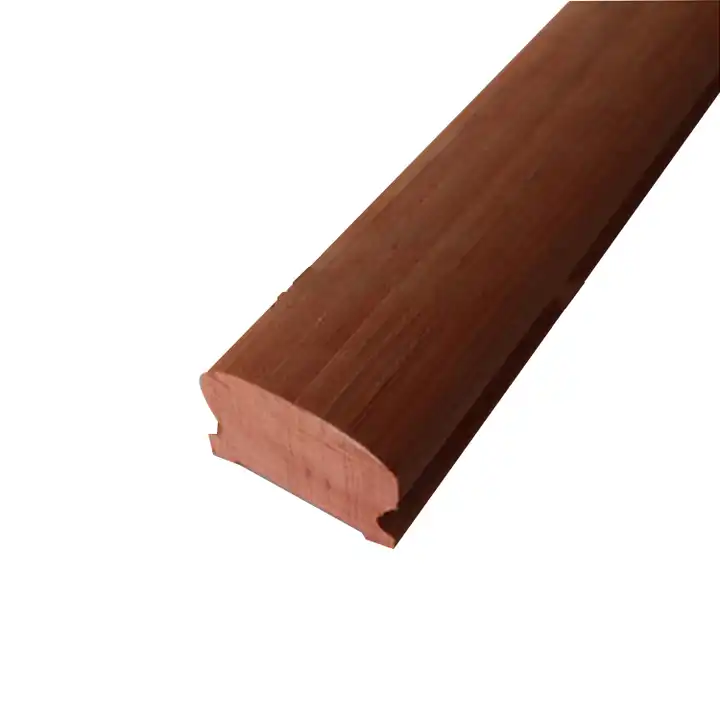This photograph features a possibly computer-generated or low-resolution image of a piece of finished wood, likely part of a railing or banister. The wood, which spans diagonally from the top right to the bottom left corner of the image, rests against a stark white background. The prominent unfinished cut at the lower left reveals a lighter, reddish wood grain, contrasting with the darker, deeper tone of the finished exterior, which exhibits black bands representing the wood grain. Notably, artifacts around the edges suggest the item was digitally extracted, possibly using a feathering tool, which contributes to the overall slightly blurry and compressed appearance of the image.